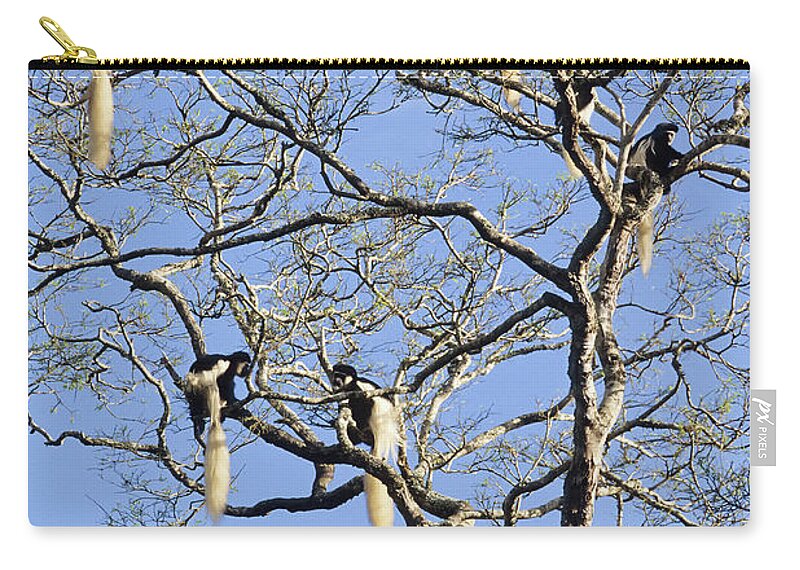This image depicts a highly detailed, photorealistic pattern on a soft robin's blue canvas bag, possibly a change purse or makeup bag, designed with a zipper at the top. The pattern showcases a series of mostly barren tree branches in shades of gray and white, adorned with minimal foliage and light touches of moss. Among these intricate branches, there are multiple black and white monkeys, potentially howler monkeys or lemurs, identifiable by their long, prehensile tails draped with powder puff-like or mullet-like fur. The scene captures at least three visible monkeys and additional tails, indicating the presence of more within the branches. The monkeys are spread throughout the tree, with two positioned in the lower section and one in the upper right corner. The background is a clear, vibrant blue sky, adding a striking contrast to the detailed branches and the monochromatic colors of the monkeys.